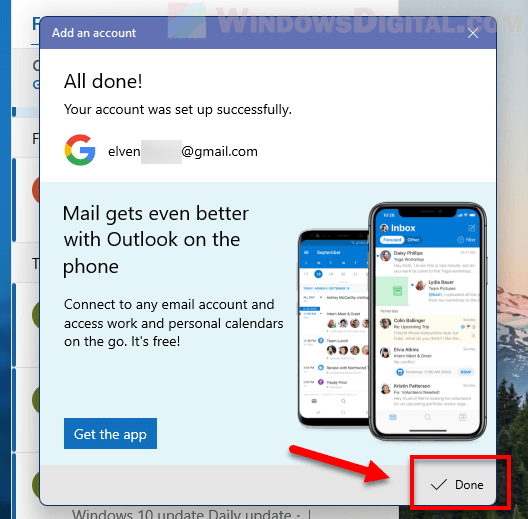This image appears to be a screenshot taken from a digital device, possibly a phone or computer. The main focus is a pop-up window superimposed over a background screen. At the top of the pop-up window, there is a partially visible purple header indicating "WindowsDigital.com". Below the header, in a prominent purple rectangle, the text reads "Add an Account."

Underneath that, there is a confirmation message: "All done! Your account was set up successfully." Notably, there is a large, colorful Google "G" icon present, indicating that the setup is related to a Google service.

Following the confirmation message, additional information suggests enhanced functionalities: "Mail gets even better with Outlook on the phone." It promotes the convenience of connecting any email account and managing work and personal calendars on the go, highlighting that it is a free feature.

The illustration within the pop-up shows two mobile phones; a smaller one in the background, and a larger one in the foreground, emphasizing mobile accessibility. Lastly, at the bottom of the pop-up, there is a red arrow pointing towards a "Done" button, which is marked with a checkmark and encased in a red rectangle, indicating the final action to complete the setup.